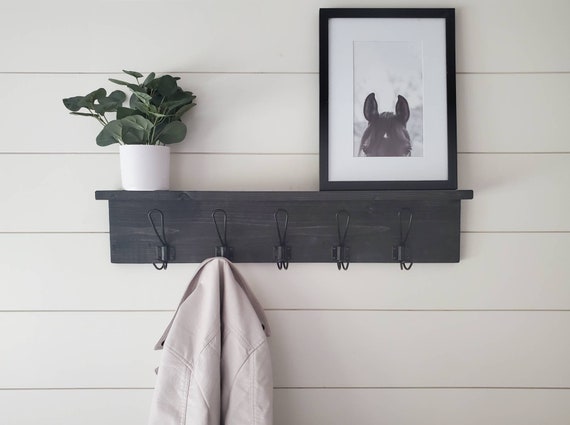This image captures a wooden mantel attached to a white wall made of vertically arranged slats. The mantel features five black-painted hooks beneath it, with a single white coat hanging from the second hook on the left. On top of the mantel, a white pot containing a plant with nearly round green leaves is positioned near the left edge. To the right side of the mantel, a framed black-and-white photograph of a horse's head is displayed. The photo highlights the horse's eyes, forehead, tuft of hair, and two pointy ears, with a distinctive white dot on its forehead. The entire setting creates a cozy, domesticated scene with a well-organized and aesthetically pleasing arrangement.